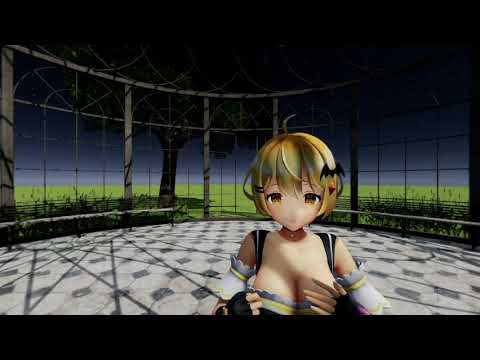In this 3D animation still, a beautifully crafted scene unfolds with intricate details. The backdrop features a striking skybox transitioning from dark blue at the zenith to a lighter shade near the horizon, setting a serene ambience over a vast, green field of light grass stretching into the distance. Directly behind the central figure stands a transparent wall made predominantly of glass panels, through which a solitary green tree is visible.

In the foreground, black and white checkered tiles form a distinguished floor pattern, possibly indicative of a gazebo area equipped with fine, arching metalwork and low bench seating. At the focal point is a young anime-style girl, likely a character from a video game, positioned just right of center on the bottom half of the image. 

She is depicted from above her bust to the top of her head, showcasing short, blonde hair that curves to her cheeks with delicate bangs and a bat-shaped hair clip. Her amber eyes are accentuated by a red choker necklace. She dons a white and yellow dress with black and white shoulder straps, presenting a bustier style top which emphasizes her ample bust and bare arms. Additional accessories include black fingerless gloves and white sleeves adorned with yellow bands.

The artistic composition harmonizes the vivacious character against the tranquil, natural scenery, blending elements of fantasy and realism in a compelling visual narrative.